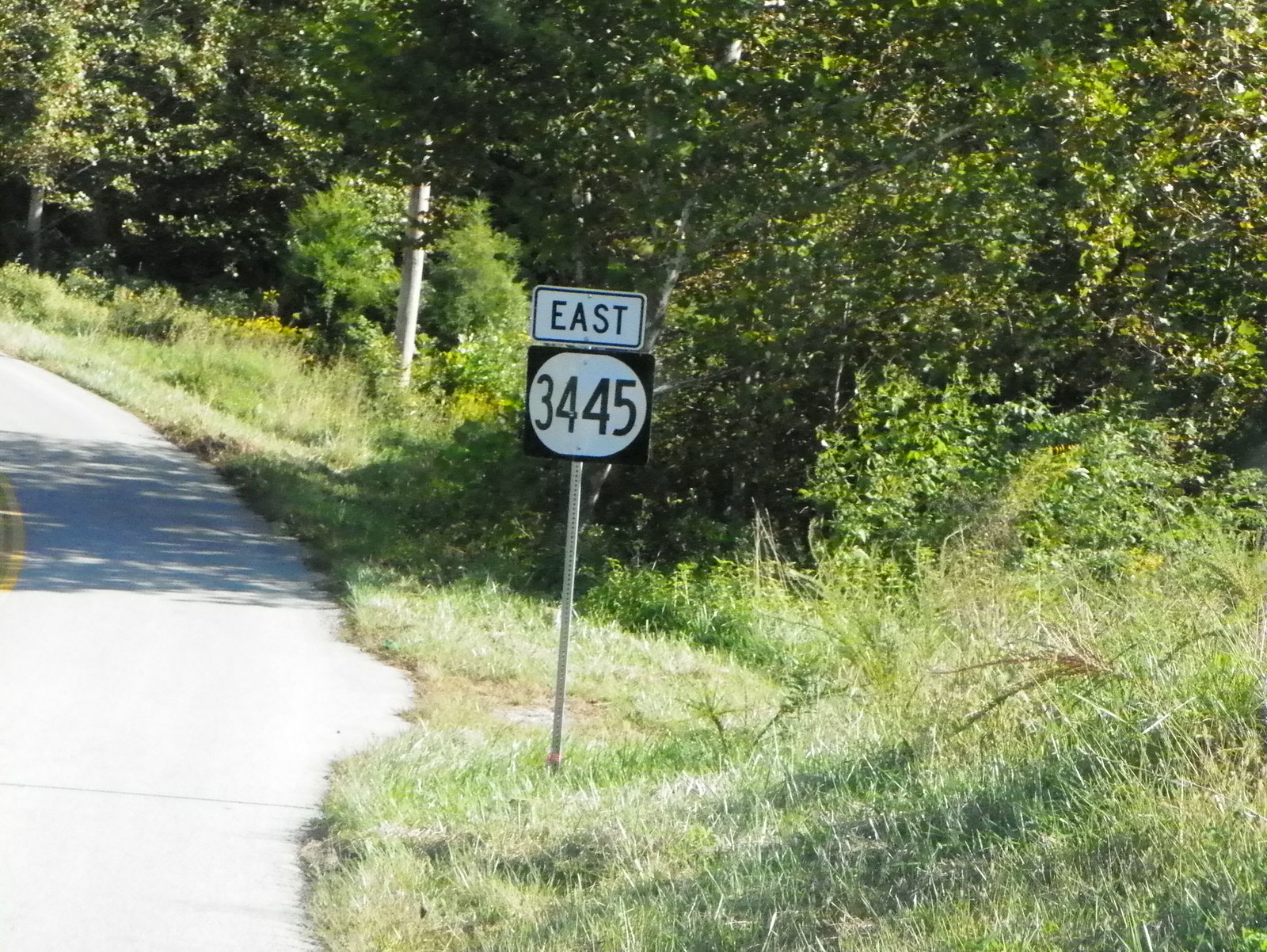A detailed highway sign is mounted on a sturdy steel pole. The lower sign is a black square featuring the number "3445" in white font. Positioned above it is an elongated rectangular sign with a white background that reads "EAST" in bold black letters. To the left of the signpost, a paved road curves gently, while the right side reveals a vast field of tall, untidy grass interspersed with a cluster of trees. Additional trees line the edge of the road, and an electrical post can be seen further down the path.